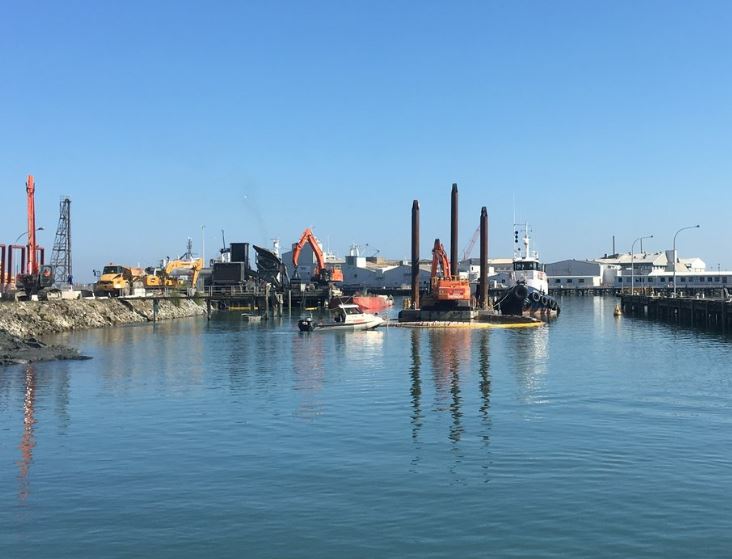This photograph captures a vibrant outdoor scene during the daytime on a large blue-hued body of water, possibly a river or a lake. In the center of the image, a variety of water vessels are visible, including both smaller and larger cargo ships, predominantly white in color. Notably, these ships are equipped with orange construction machinery. Moving towards the left side of the photograph, a road is visible with larger construction vehicles positioned along it. On the right side, there is a wooden dock or pier area. At the forefront of the image, white buildings are discernible. The sky above is a clear blue, enhancing the overall bright and bustling atmosphere of the scene. The photograph is almost square in composition, with the water body situated towards the bottom and the sky occupying the top part of the frame. The overall setting is unmistakably outdoors during daytime.